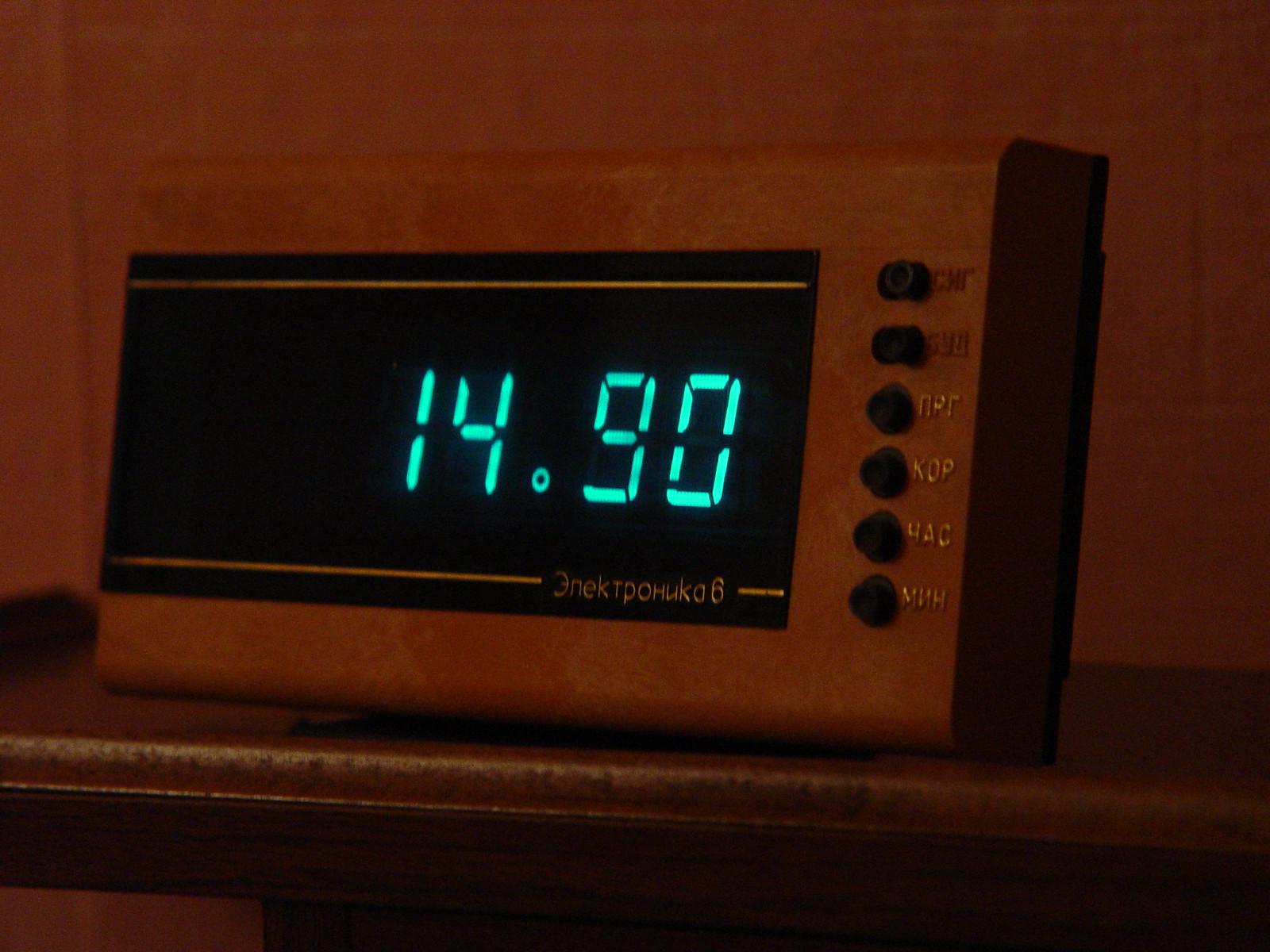A photograph of an old Russian digital clock resting on a round-edged, wooden table in a dimly lit room. The room and the clock exhibit various shades of brown, contributing to the overall warm, subdued ambiance. The clock features a vintage digital display with light green numbers, showing the time "14:90." Above and below the numbers, there are gold lines, with a portion at the bottom right corner interrupted by some Russian text and the number "6." To the right side of the clock are six small black buttons, with raised golden Russian letters adjacent to each button. The photograph captures the nostalgic charm of the clock, though the low lighting might slightly distort the actual colors.